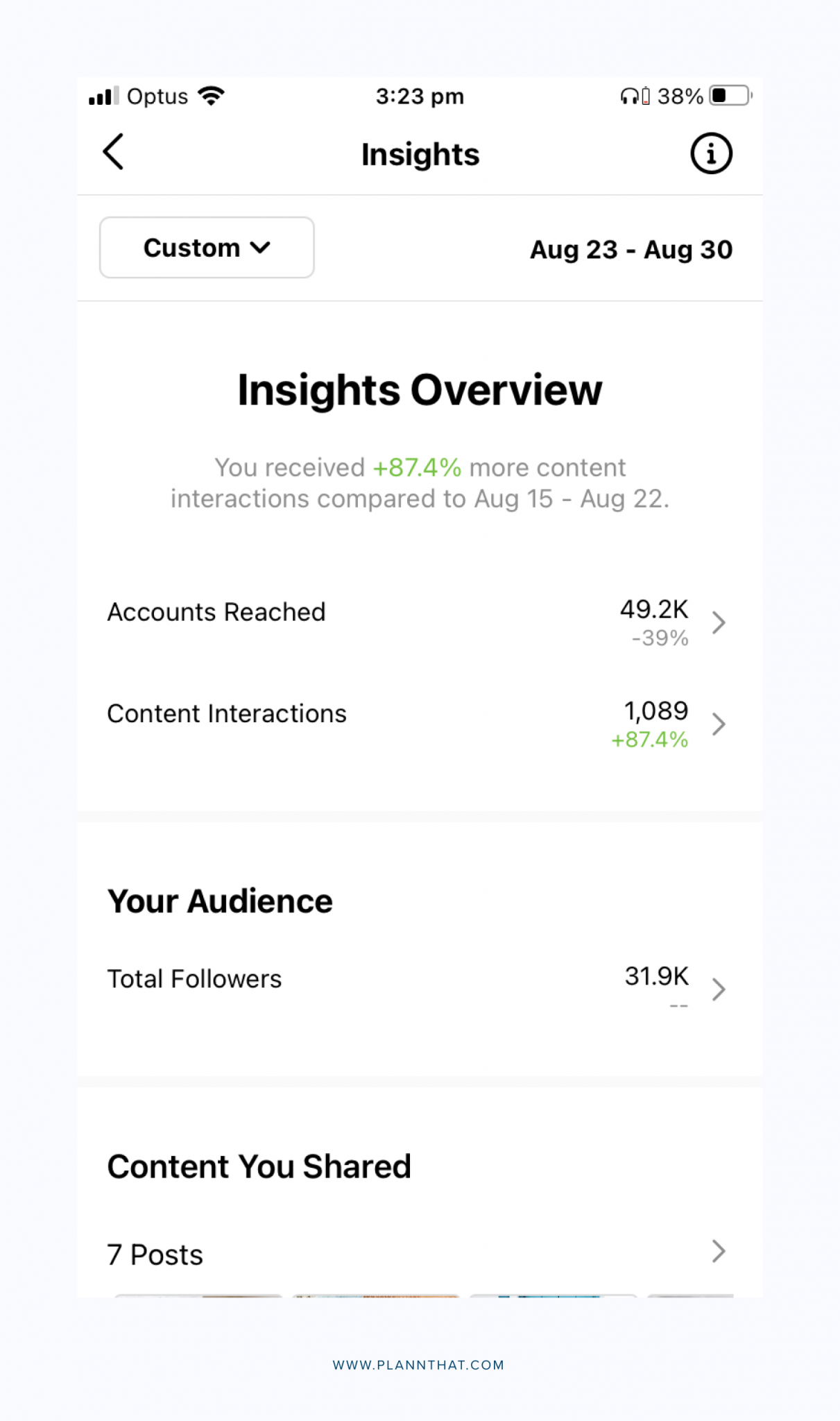### Detailed Image Caption:

The screenshot features an insights overview page on a website, depicted against a completely white background. The main content of the page, consisting of large dark text, is positioned towards the center and upper center of the screen. The header at the very top of the screen displays standard smartphone interface details. On the upper left corner, the mobile carrier "Optus" is indicated, accompanied by three or four vertical bars, signaling the network strength. On the opposite side, there are three arcing upward lines representing the Wi-Fi symbol.

Centrally located in the top bar, the current time is displayed as 3:23 p.m. The right side of this bar shows four distinct icons sequentially: a headphone icon, a battery charge icon, a low charge warning labeled "38%," and a partially charged battery icon.

Directly beneath this bar is a prominent header labeled "Insights," with a back arrow icon on the far left and a circular icon with a lowercase "i" on the far right, suggesting important information is accessible by clicking it. Below this, there is a customized period dropdown button labeled "Custom" on the left, paired with a date range indicator, "August 23rd to August 30th," on the right.

Next, the text "Insights Overview" introduces the main content area. Beneath it, a grayed-out comment states, "You received 87.4 more content interactions compared to August 15th to August 22nd," with the numerical value "87.4" highlighted in green.

Following this, two main metrics are presented: "Accounts Reached," listed as 49.2k with a grayed-out decline of -39% below it, and "Content Interactions," noted as 1,089 with a green-highlighted increase of +87.4%.

The subsequent section titled "Your Audience" is in black text, under which "Total Followers," accounting for 31.9k, is shown with a clickable arrow for additional information. Concluding the main body, the section "Content You Share" states "7 posts" and includes another arrow for more details.

At the very bottom of the screen, the URL www.planandthat.com is displayed.